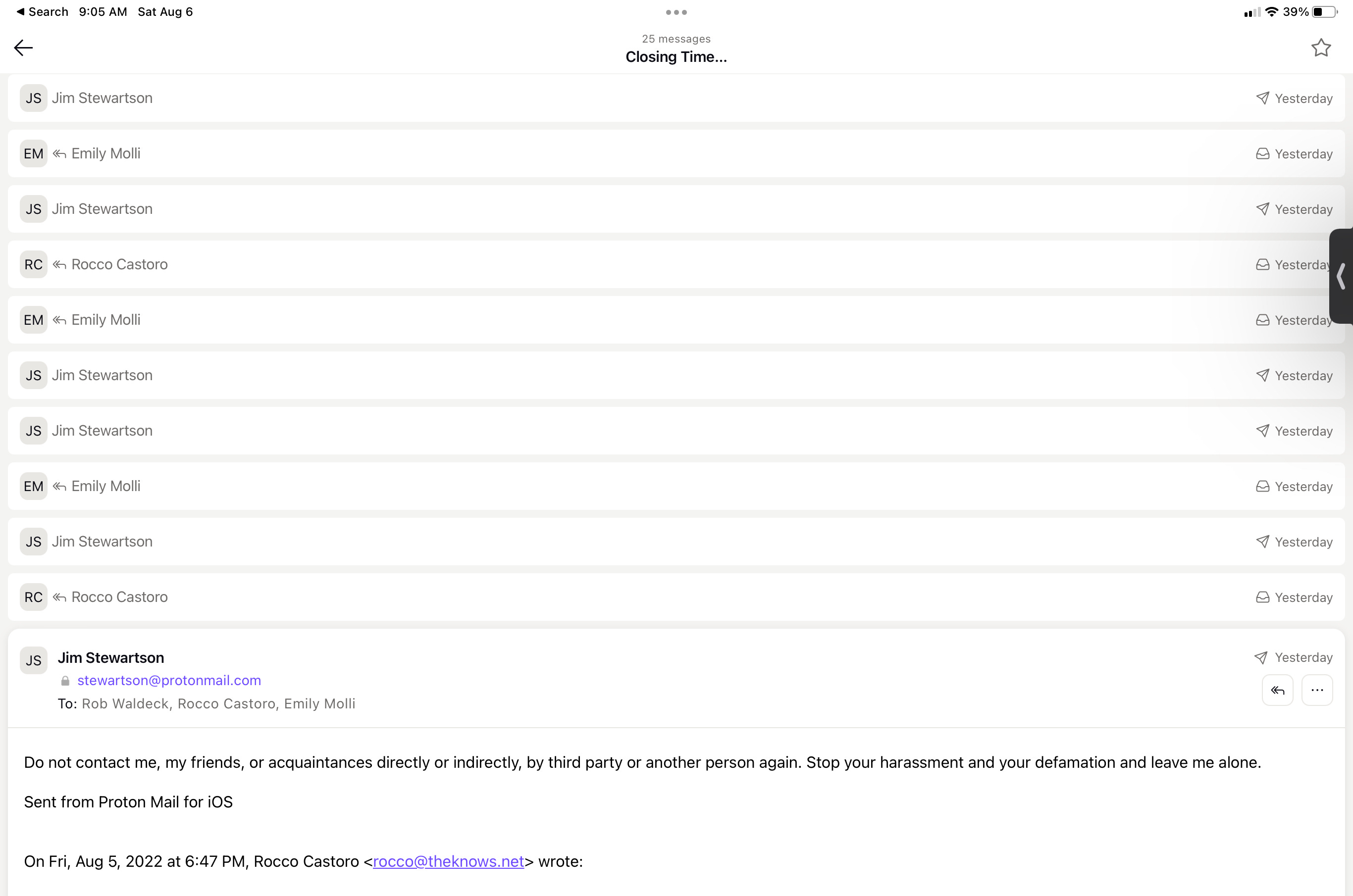In the image, there's a detailed screenshot of what appears to be an email list with various elements. At the top, there's a date and search box saying "9 a.m. Saturday, August 6." On the far right, it indicates the mobile signal strength and battery percentage, showing 39%. Below this, there's an arrow pointing left with the text "25 messages closing time" and a star icon to the right.

The main section contains a list of names, including Jim Stewart, Emily, Molly, Rocco Castoro, and repeated instances of Jim and Emily. To the right of each name, the word "yesterday" is displayed, and some names are accompanied by triangle and printer icons. 

At the bottom, Jim's email address is visible. Below that, there is a small black text note stating: "Do not contact me, my friends, or appointments directly or indirectly by third party or another person. Stop your harassment and your defamation and leave me alone," followed by "Sent from Proton Mail for iOS." The date at the very bottom shows "Friday, August 5, 2022, at 6:47 p.m." and it is from Rocco.